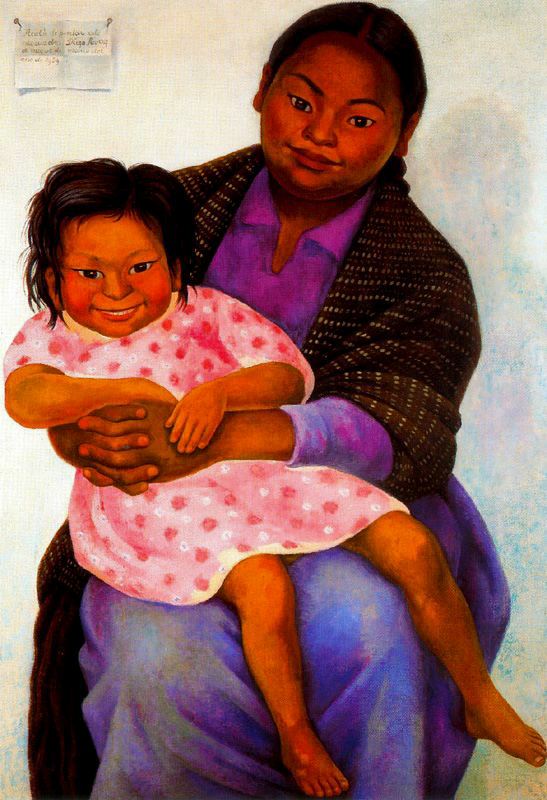The image is a stylized painting of an African-American mother and daughter. The mother, wearing a brownish dotted jacket over a purple dress, sits on an unseen chair against a white background. She has short black hair and her head is slightly cocked to the left. Her expression is neutral as she gazes directly at the camera. The young daughter sits comfortably on her lap, dressed in a pink and red polka-dotted dress that reaches just above her knees. The girl, with medium-length dark hair and pronounced, cheerful smile showing her teeth, contrasts with the mother's more solemn demeanor. Both share the same large almond-shaped brown eyes. In the upper left-hand corner of the painting, there is a note pinned to the wall with writing in an unknown language, although the specifics of the text are illegible.